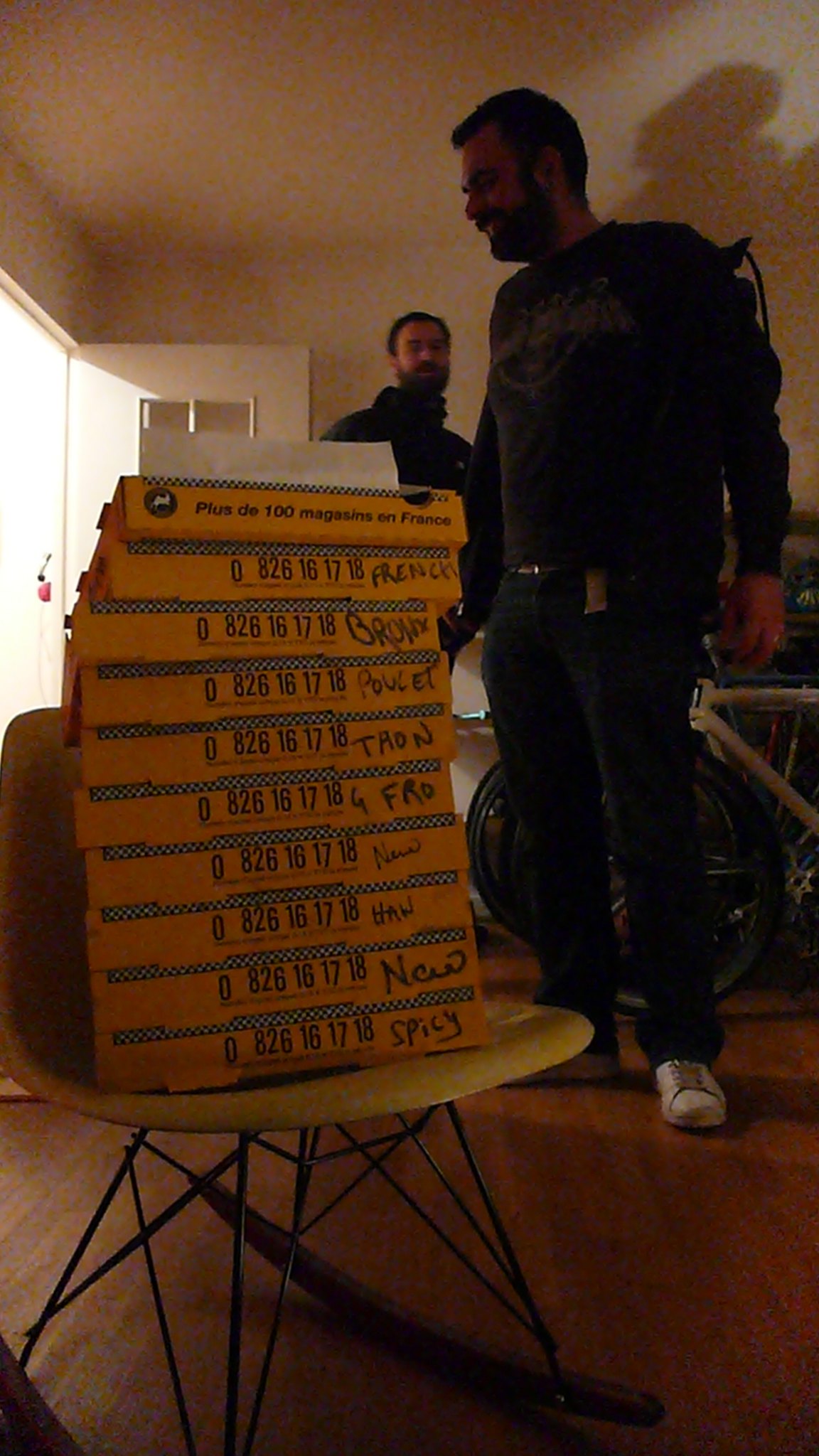In this photograph, two bearded men are captured in a dimly lit room with an open door that allows daylight to pour in. Both are dressed in dark clothing; one is in all black, while the other sports a black hoodie. In the foreground, there is a table with ten orange pizza boxes, neatly stacked. Each box displays an identical number sequence—0 826 16 17 18—possibly a French phone number. The boxes, reminiscent of Little Caesar's packaging, feature various handwritten labels such as Spicy, New, Han, Naw, Forfro, Tron, Pousset, Bronx, and a top label indicating "over 100 magazines in French." Additionally, a black-wired chair is partially visible beneath the stacked boxes. There are bicycles in the background, adding to the room's cluttered appearance. One of the men appears closer to the pizzas, casting a shadow on the wall, while the other stands further back, partially obscured. The scene's lighting and the open door suggest they’ve just brought the pizzas inside.